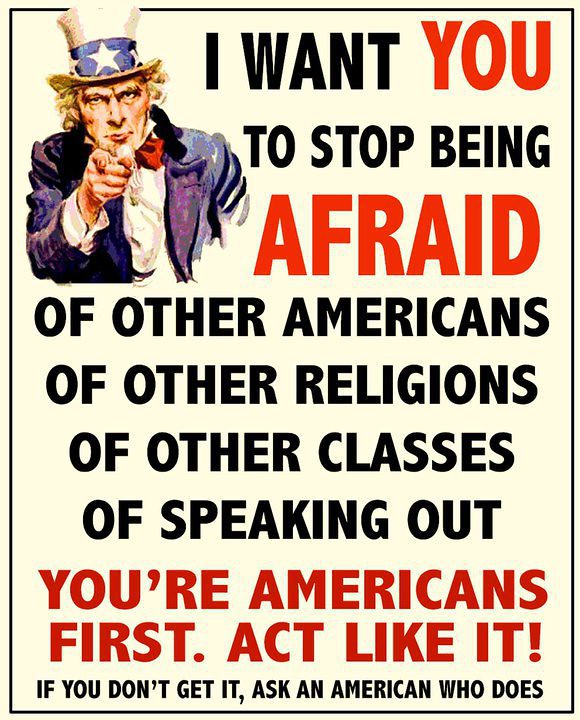The image is a rectangular poster with a cream-colored background and a black border. In the top left corner, it features the iconic image of Uncle Sam pointing his right finger directly at the viewer. He is wearing his characteristic tall top hat, which is white with a blue stripe and a white star, a blue coat with a white undershirt, and a red bow tie. His hair is sticking out slightly from under the hat, adding to his distinctive appearance. Below the image is bold text in red and black that reads: "I want you to stop being afraid of other Americans, of other religions, of other classes, of speaking out. You're Americans first. Act like it. If you don't get it, ask an American who does." The phrase "afraid" as well as "You're Americans first. Act like it." are particularly emphasized in bold red letters. The poster calls for unity and courage among Americans, urging them to overcome fears related to differences in religion, class, and the act of speaking out.